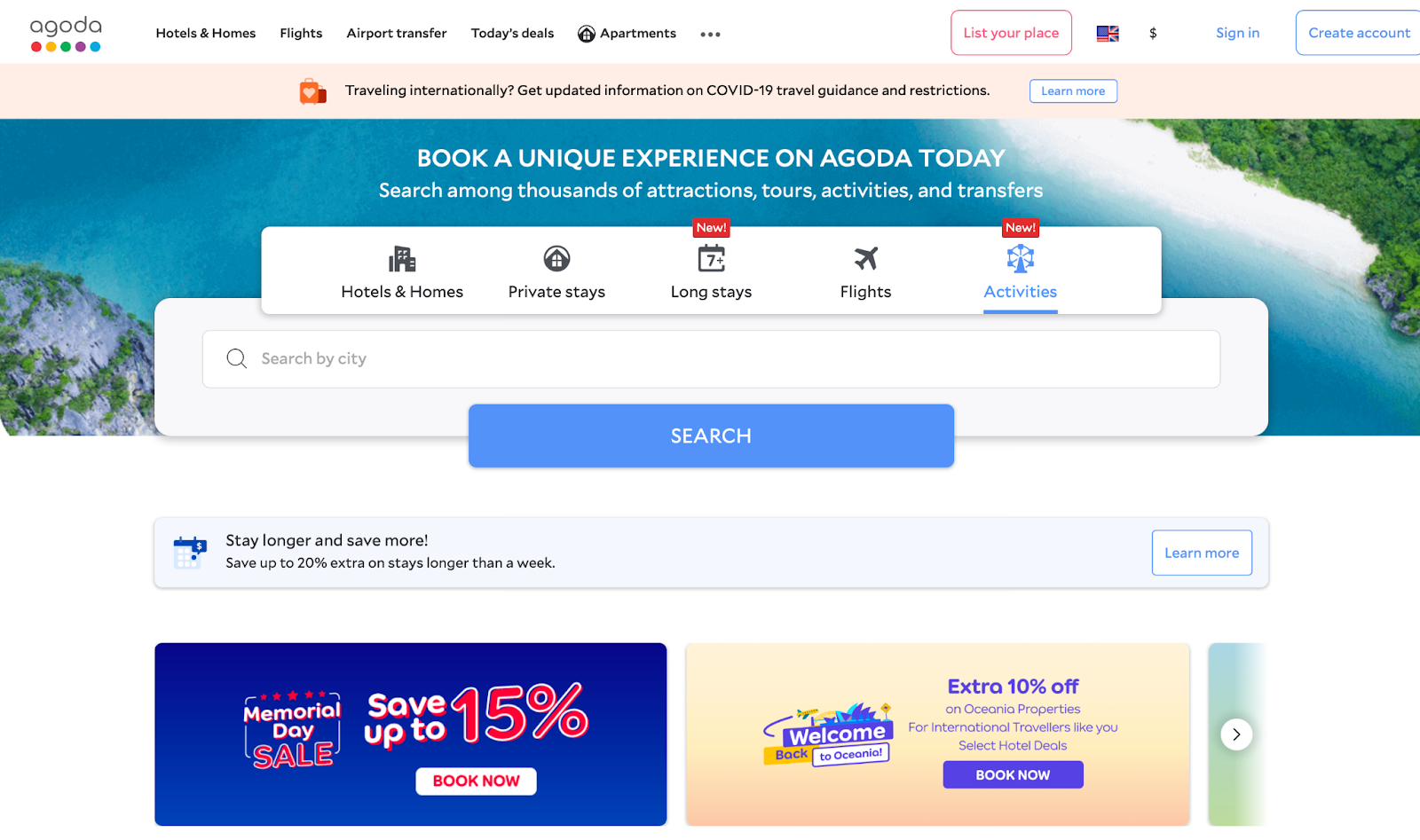The image is a left-to-right horizontal advertisement, commonly seen on a computer, sent via email, or displayed on a webpage, smartphone, or smart device. The background is plain white, emulating a computer screen. 

At the top of the image, the brand "Agoda" is printed in black. Below this, there's a row of differently colored circles. From left to right, the text reads: "Hotels and Homes," "Flights," "Airport Trips," "Today's Deals," and "Apartments." Following this is an ellipsis indicating more options.

A little further along, in red text, it says "List your place," accompanied by icons of a flag, a dollar sign, and blue-text options "Sign In" and "Create Account."

Next is a peach-colored rectangular box featuring a shopping bag icon and a message about international travel. It urges users to get updated information on COVID-19 travel guidance and restrictions, with a prompt to "Learn More."

Below this, there is a beach-themed background depicting an aerial view of the ocean, sand, and trees. The text encourages users to "Book a unique experience on Agoda today, search among thousands of attractions, tours, activities, and transfers." 

There are buttons for "Hotels and Homes," "Private Stays," "Long Stays," "Flights," and "Activities." Users can search by city using the input field accompanied by a blue "Search" button. There is also a slogan "Stay longer, save more," with a link to "Learn More."

At the bottom, the advertisement features promotional offers: a "Memorial Day Sale" with savings up to 15%, options to "Book Now," and an offer for "Welcome to Oceana," giving an extra 10% off Oceana properties.